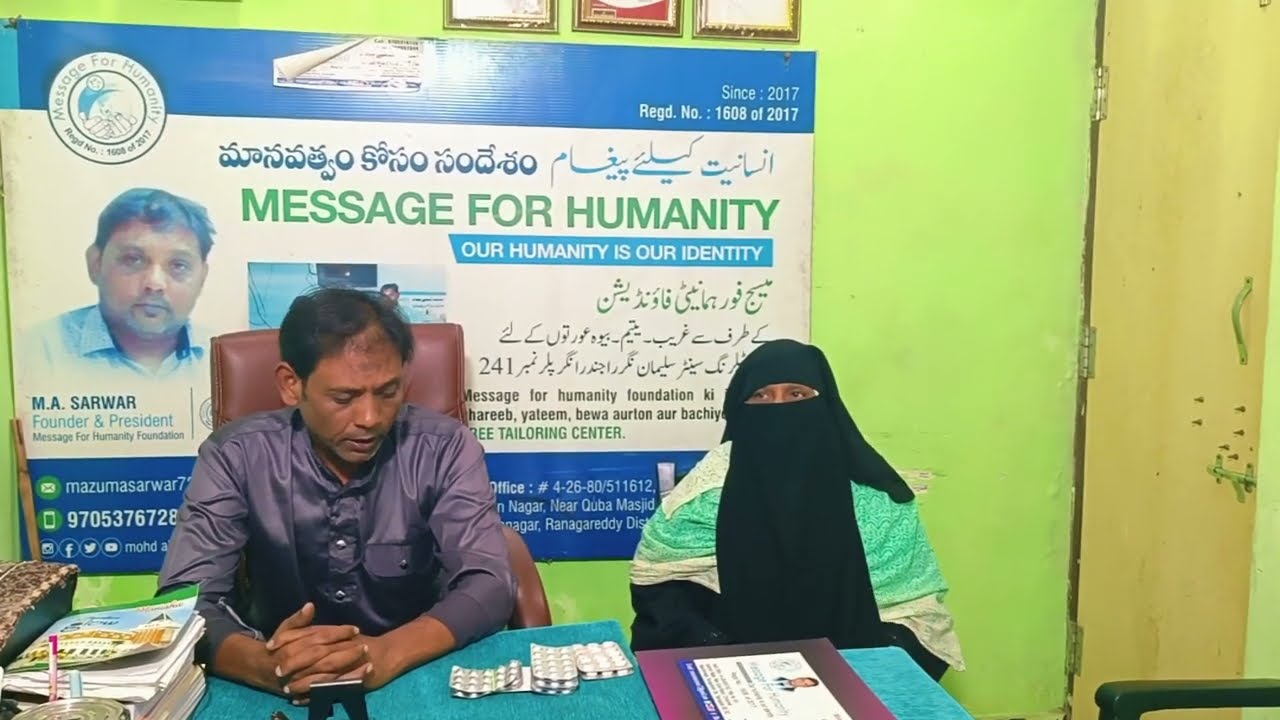In this image, we see a man and a woman seated at a table, positioned centrally within the frame, appearing to be part of an indoor press conference or similar event. The man, located on the left, is wearing a shiny purple dress shirt with silver snap buttons, seated in a brown leather chair. He has black hair that is balding at the center and is looking down at various items on the table, which include packages that resemble pill containers. The table is draped with a blue cloth. The woman next to him on the right is dressed in a black burka with green accents, covering her entire face except for her eyes. She is looking off to the side. Behind them, a large green sign with a photograph of the man and text in both English and a foreign language reads: "Message for Humanity. Our humanity is our identity. M.A. Sarwar, founder and president." The scene is colored with shades of green, tan, white, blue, purple, black, and pink, setting a formal and focused atmosphere.